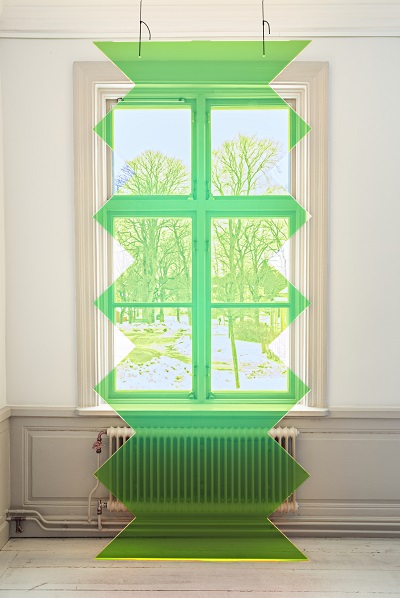This photograph captures an indoor scene focused on an eye-catching green vertical art piece suspended in front of a white framed window. The art, resembling a somewhat translucent window shade or abstract green Christmas tree, features prominent chevron or zigzag patterns along its sides. The structure, made from either acrylic or glass, has a distinctive rectangular window with a cross in the center, through which vibrant green trees are visible, giving a surreal, filtered view of the outdoors. This hanging piece is attached to the ceiling by two strings or ropes and extends downward, with its lower portion spilling onto the hardwood floor. The room's decor is in muted tones, with white walls and gray wainscoting, complemented by an off-white or gray radiator below the window. The overall ambiance of the room is neutral, allowing the striking green art piece to dominate the scene.